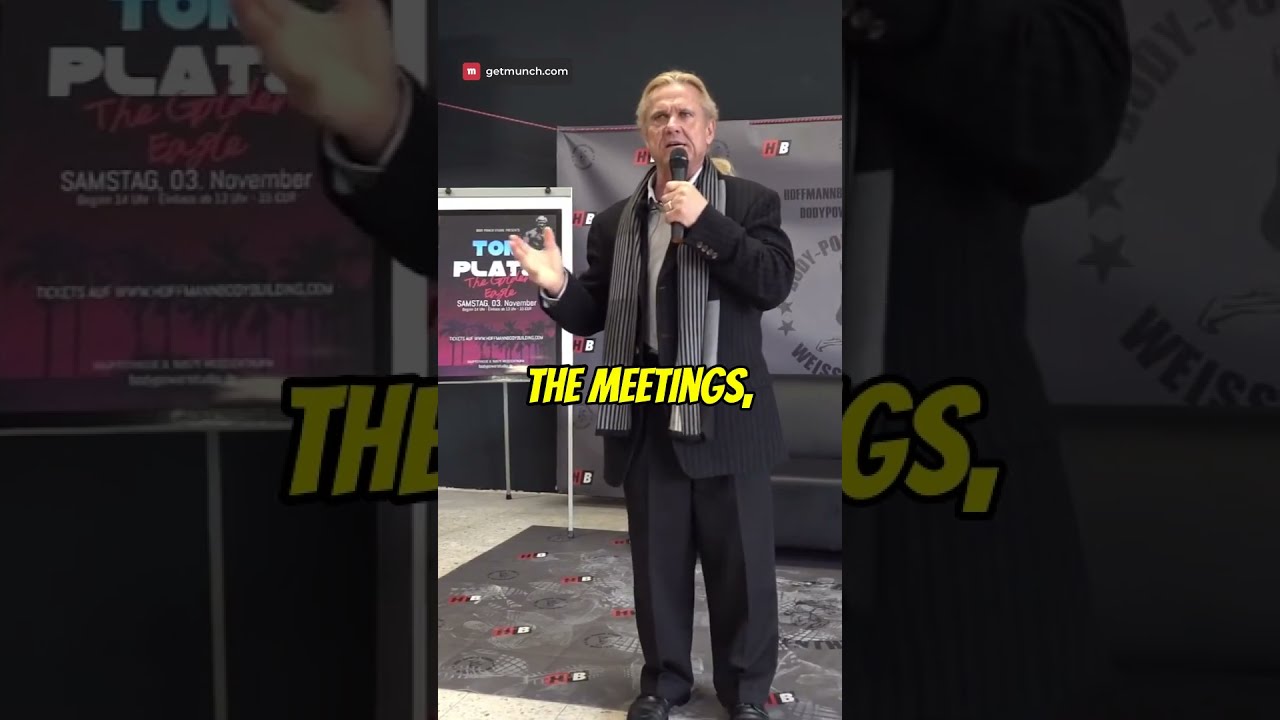In this detailed photograph, a man with blonde hair streaked with gray, pulled back into a ponytail, is standing on a yellow linoleum floor that partly covers a short gray-red-and-white carpet. The man is dressed in a baggy, dark gray suit with black slacks and black shoes, complemented by a long black-and-white vertically striped scarf that hangs down to his waist. He has saggy jowls and a notable large ring on his ring finger. With a serious expression, he faces the viewer, holding a microphone in his left hand up to his face while his right hand gestures outward, possibly delivering a presentation or addressing an audience.

Above him, yellow text overlaid reads "the meeting." Behind him is a somewhat obscured banner that seems to read "T-O-P-L-A-T" and another sign to his left that partially reads "Tony" due to his extended hand blocking it. The background includes additional signs with lettering that is largely cut off or partially hidden, adding to the enigmatic and professional atmosphere of the scene.